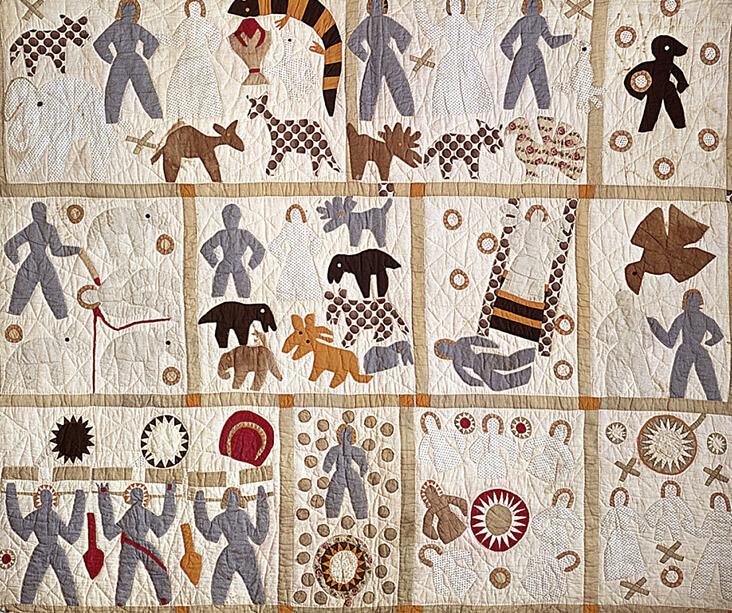The quilt in the image is an intricately designed textile featuring a variety of scenes and figures that give it an almost Egyptian or American Indian aesthetic. The quilt is divided into multiple square panes, each adorned with unique images. It predominantly uses a color palette of creams, light browns, medium browns, faded blues, black, white, red, gold, and bronze. The quilt is bordered with bronze, clearly separating each pane. 

Key details include:
- Various figures in different hues, particularly notable are blue people, a lady in a white polka-dotted dress, and a black figure holding a round cylindrical shape.
- Several scenes depict animals such as birds, zebras, camels, dogs, elephants, and possibly tigers and salamanders.
- Specific panes show a brown bird hovering over two people, a scene indicating a death and an angel, and three men holding up blocks.
- One pane features a blue man surrounded by round circles, while another displays women with horseshoe-shaped hairstyles in polka-dotted attire.
- The quilt also includes numerous X patterns and a sun dial design in one of the frames.
- Overall, the detailed and varied imagery, alongside the use of color and pattern, suggests it could be a childhood quilt, rich with symbolic meaning and artistic expression.